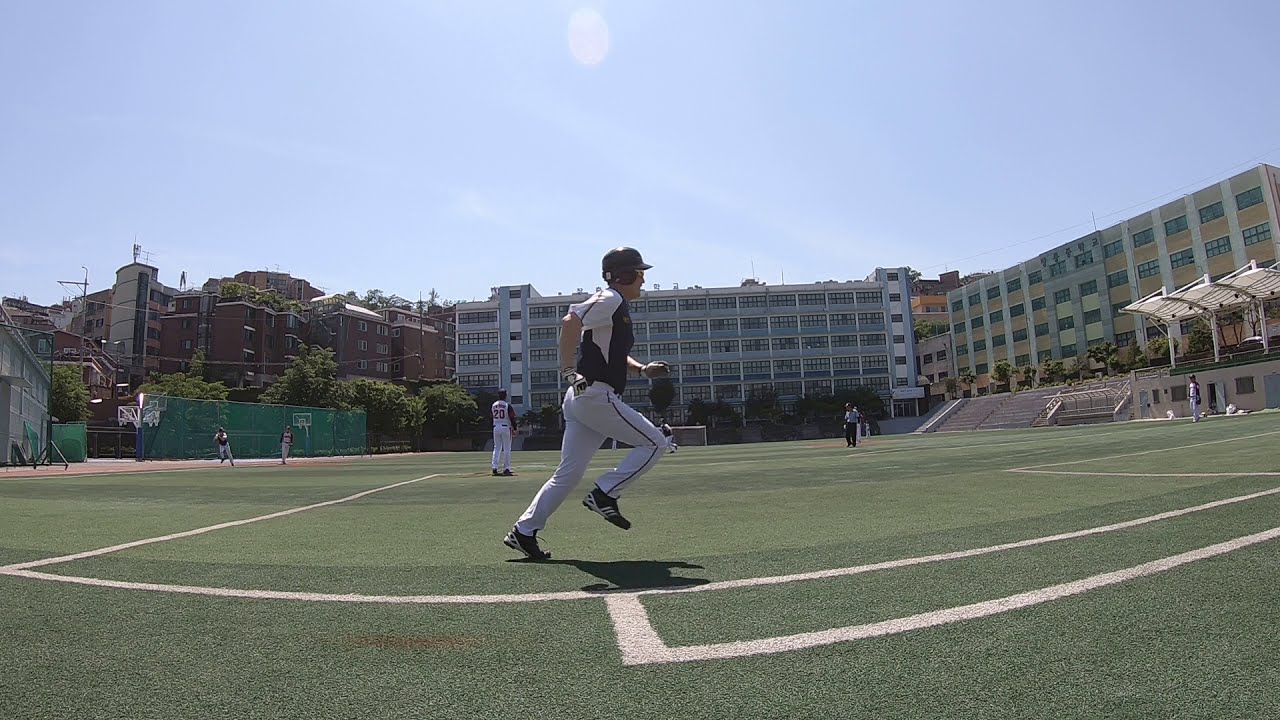The photograph captures a vibrant baseball scene with a central baseball player, dressed in a blue and white uniform with the number 20 on the back, sprinting across an artificial turf field. The player, wearing a helmet, is possibly mid-practice or celebrating a run, surrounded by teammates in similar uniforms scattered across the field. The setting is more reminiscent of a multi-use sports field, with visible white stripes and possibly soccer markings, rather than a traditional baseball diamond.

In the background, an L-shaped, six-story building, possibly an apartment complex, looms large, composed of brown brick and flanked by a gray structure nearby. Additionally, there are several basketball hoops and green chain-link fences indicating the multi-sport usage of the area. Stadium seats line one side of the field, though they appear empty, reinforcing the idea that this is a practice session. The entire scene is bathed in daylight, with the sun shining brightly under a clear blue sky, highlighting the vibrant, green artificial turf.